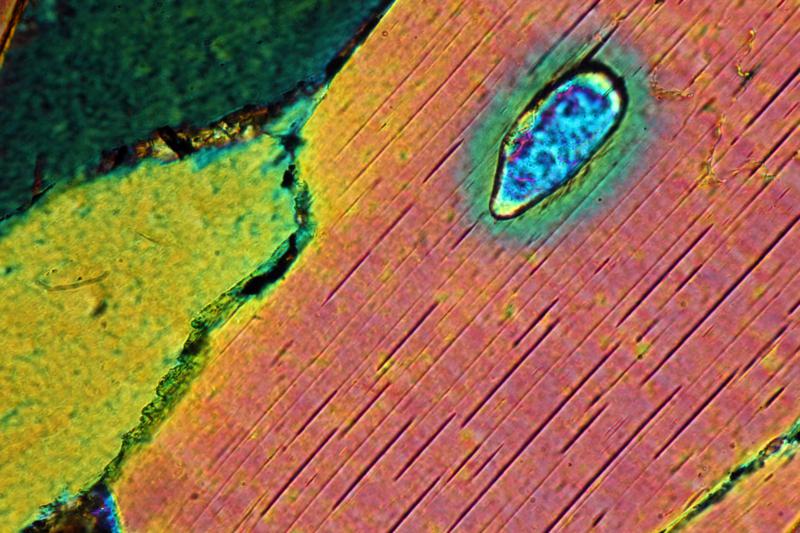The image, oriented in landscape, appears to be a colored or dyed photograph of something viewed under a microscope. Predominantly covering the right side and extending diagonally towards the left, the picture features a pinkish, striated design interspersed with dark lines and occasional yellow tinges. In the upper left corner, there is a dark green area lightly tinged with yellow, bordered distinctively from adjacent sections. Below this and occupying the bottom left is a bright yellow region scattered with green specks. 

Centrally within the pink expanse, slightly off towards the top right, a cell-like structure stands out, characterized by a black outline encapsulating blue and purple interiors, and surrounded by a greenish-yellow aura. From the bottom right corner, another green and yellow streak meanders through the pink area before disappearing off the image’s lower edge. The interplay of colors and shapes, combined with the intricate boundary lines, contributes to the complexity of this microscopic landscape.